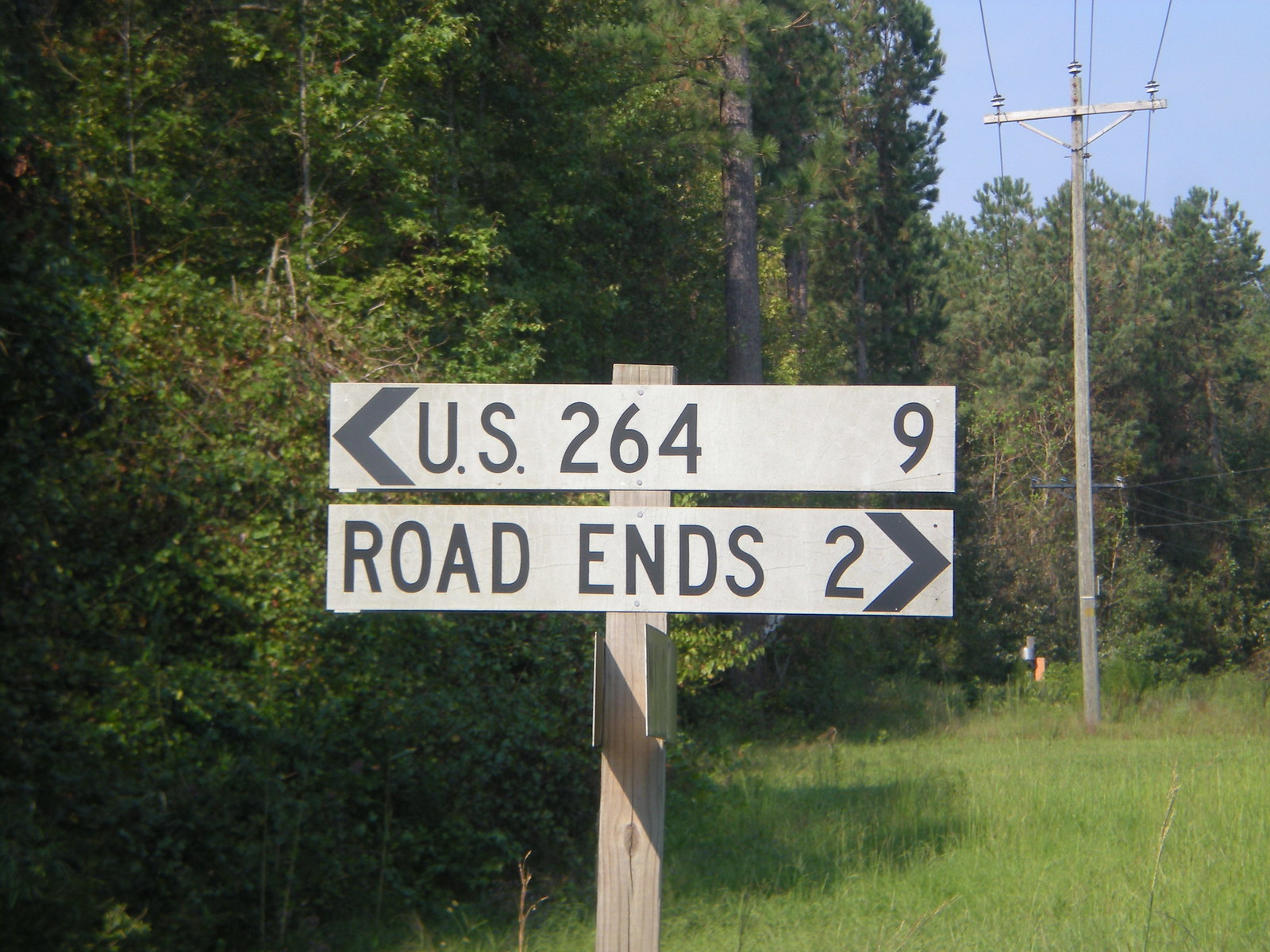In this daytime color photograph, a pair of white rectangular signs with black lettering are mounted on a weathered light brown wooden post, set amidst a country landscape with very high grass or weeds along the road. The top sign features a black chevron-styled arrow pointing left, the text "U.S. 264" followed by a large numeral "9" positioned on the right. Below it, another sign states "ROAD ENDS 2" with a chevron pointing to the right. Dominating the right background is a tall gray power pole, adorned with insulators and carrying multiple power cables towards the camera. The scene is framed by a dense tree line featuring a mix of deciduous and pine trees, extending from the left side to the back right, bathed in the light of a beautiful summer day. An orange gas tag sticker is visible on the pole, and a patch of blue sky peeks through in the top right corner, enhancing the serene rural setting.